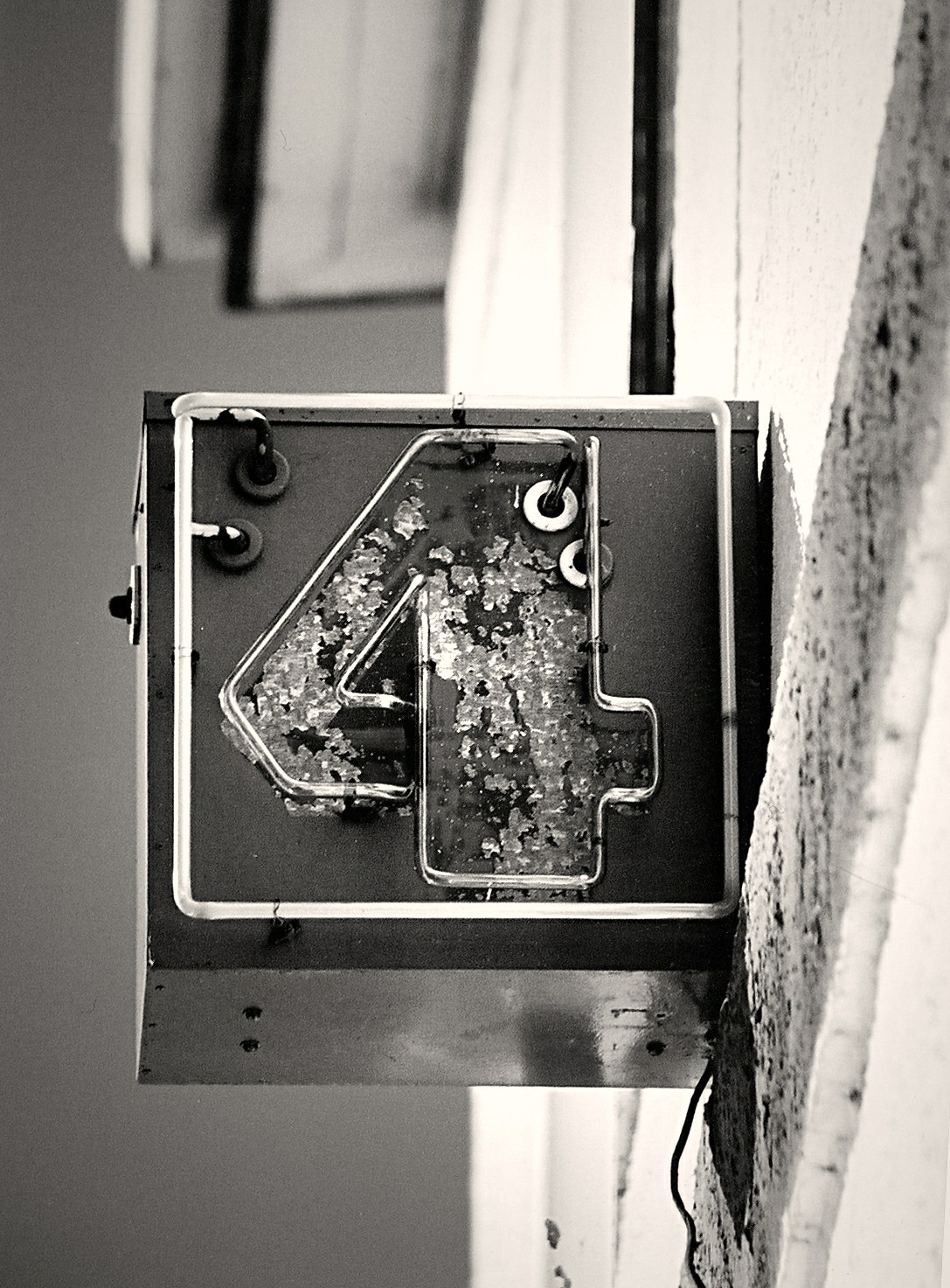The black and white outdoor image is taken from a low angle, looking upwards toward the side of a building. The building's facade features a mix of materials, possibly stone and wood, painted white and trimmed with black. Dominating the scene is a metal sign attached to the building, which appears to be aged and damaged. This square-shaped sign, outlined with black hooks, prominently displays a neon number four, which is surrounded by a broken glass covering and rusting edges. The front of the sign houses a small black switch that might have been used to turn it on. Above the sign, a white lower roof with black trim and a higher white roof are visible, framing a grayish sky that enhances the contrasting architectural elements.